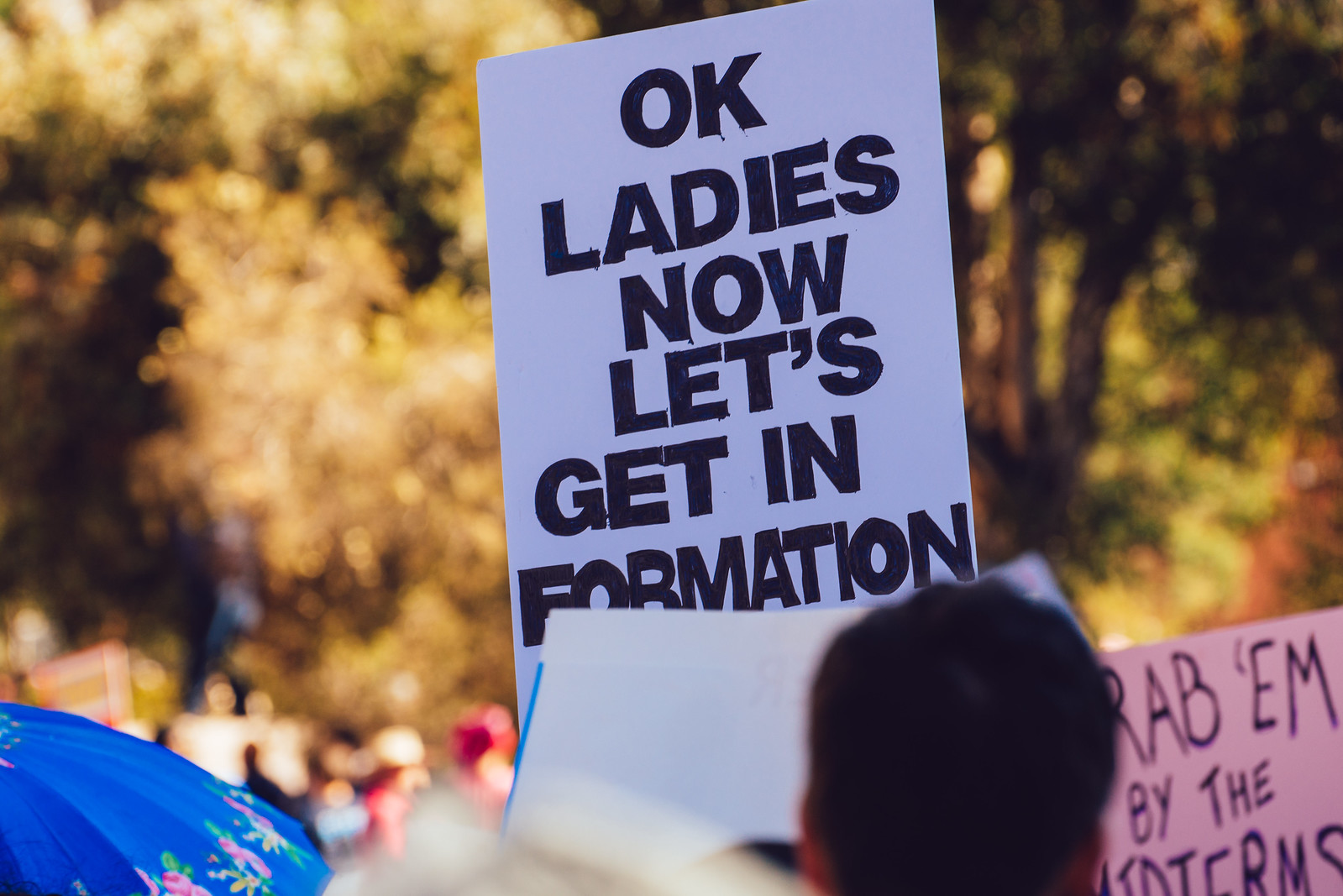This color photograph captures an outdoor event, likely a protest or rally, bathed in daytime sunlight. The background features trees with a yellowish tint, suggesting a fall setting, and blurry figures of people. These blurred individuals, along with the sunlight filtering through the leaves, emphasize the lively yet indistinct setting. In the foreground, the back of a dark-haired person's head is prominently visible, with a detailed blue floral umbrella in the lower left-hand corner. To the lower right-hand corner, a pink sign with black text is partially legible, showing the words "grab them by the" and an obscured word. Dominating the center of the image is a white banner with bold black text proclaiming, "OK, ladies, now let's get in formation." The overall scene suggests a vibrant and dynamic organized gathering.